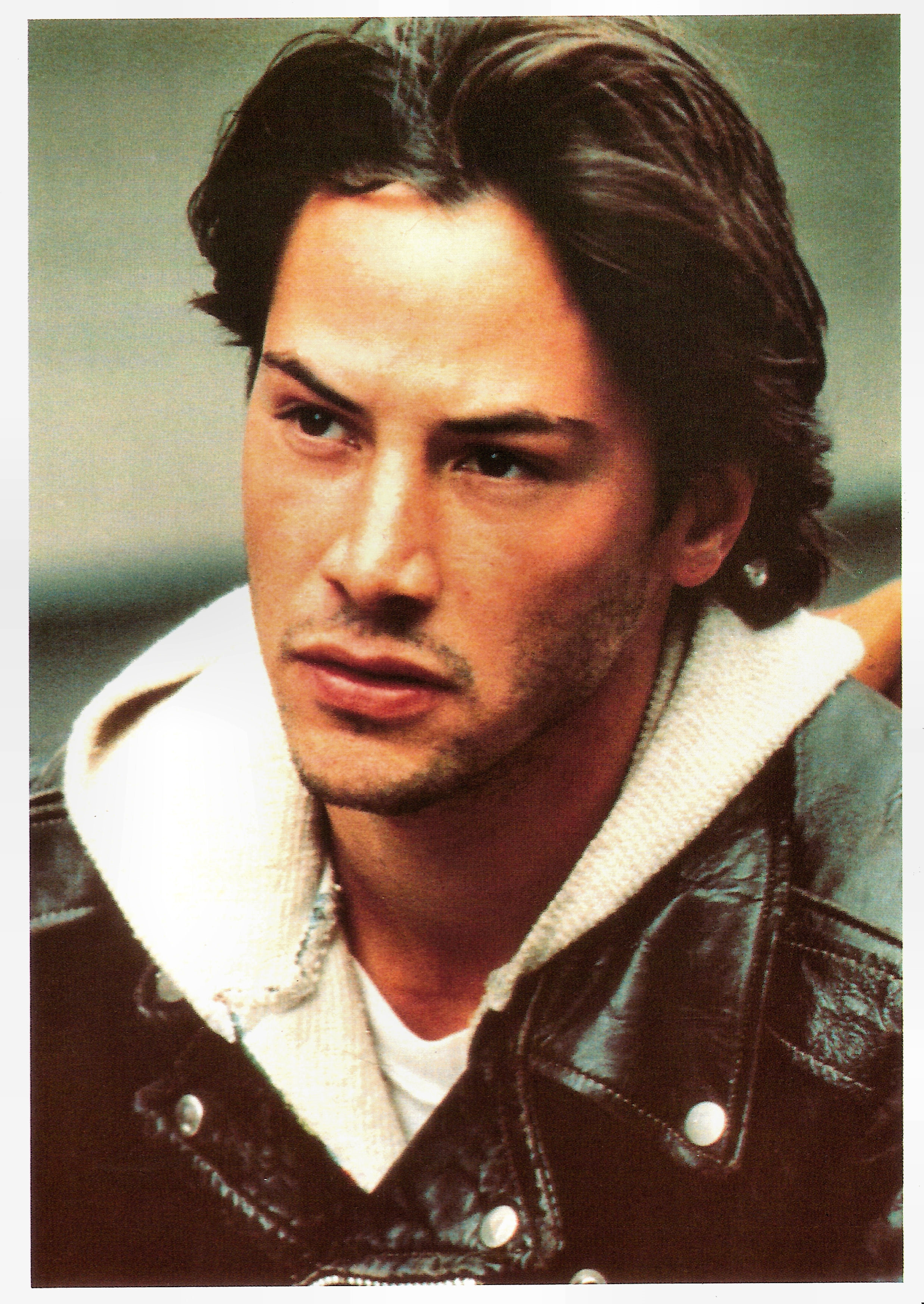This image is a vintage portrait of a young Keanu Reeves. He is depicted wearing a shiny black leather jacket with silver snaps and buttons, over a white hoodie which has a white t-shirt underneath. Keanu’s complexion is fair with a peachy tone, and his hair is dark brown, straight, slightly wavy, and medium-length, styled back with some volume at the top. The portrait captures him from the chest up, with his head almost centered in the frame. Keanu has a thoughtful and quizzical expression, looking off to his right into the distance rather than directly at the camera. There is a slight hint of facial hair, namely a light mustache. The background of the image is blurred with a grayish white tone, adding to the timeless quality of this classic photograph.